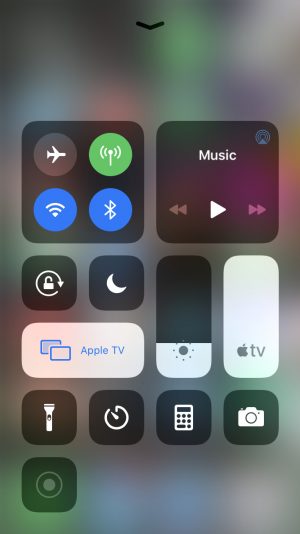This screenshot from an iPhone captures the Control Center interface, showcasing various quick-access settings and tools. Dominating the top segment, we find connectivity icons including Airplane Mode (represented by an airplane icon), Wi-Fi, and Bluetooth settings grouped together for easy access. Adjacent to these controls is the music control widget, which includes a play button beneath a grey music note icon, allowing for seamless media playback.

The middle section features several toggle buttons: the screen rotation lock, symbolized by a rotate icon, and a Night Shift mode, indicated by a moon icon, which adjusts the display's color temperature for better night viewing. Brightness control is represented by a slider, and the Apple TV mirroring function—distinguished by an Apple TV icon—enables the mirroring of the phone display to an Apple TV.

The bottom segment includes additional utilities such as a flashlight icon, a timer app shortcut, a calculator app shortcut, and a camera app icon for quick access to photography functions. Notably, there is an icon identified as "Not an iPhone" indicated by a circle, which likely signifies an external device or setting not specific to an iPhone.

The very top of the interface contains a downward-pointing arrow, hinting at a drop-down menu for more options. The background of the entire Control Center is blurred, providing focus on the icons while still maintaining a sense of context.